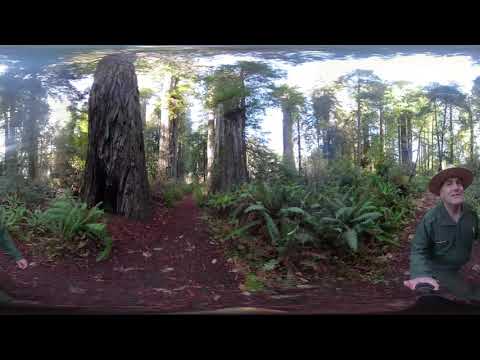In this vibrant, sun-dappled tropical setting, a middle-aged man dressed in a green suit, reminiscent of a park ranger or someone on a safari, stands on the far right of the image. He is wearing a light-colored straw hat and seems to be smiling at the camera. While no specific badges are visible, what might be a name tag is seen on his right pocket. Surrounding him is a lush jungle scene filled with more than ten large trees that form an almost impenetrable canopy, allowing filtered sunlight to pierce through. The ground beneath is a mix of red clay-like dirt and scattered leaves, with some ferns and yucca-like plants dotting the forest floor. Despite some picture distortion at the very top where the sun shines through the tree leaves, the overall atmosphere exudes the serene beauty of a sunlit clearing deep within a tropical forest.